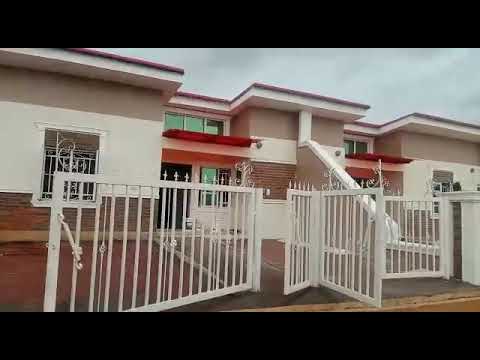The image captures the front view of a residential building, possibly townhomes or condominiums, characterized by a modern architectural style. The structure is divided into two symmetrical units, each featuring a white metal fence with small spikes along the tops, partly open in multiple sections, revealing partial views of both homes. The building itself is primarily white with beige or light brown trimmings, and the lower half is constructed from red brick. Each unit has a flat roof and a prominent bright red awning over the entryway. The facade includes various square windows and a sliding glass door, with both the awnings and windows indicative of coordinated design elements. A wall separates the two identical units, creating a sense of division while maintaining architectural harmony. The image, taken during the day, also includes a expanse of sky at the top, further situating the scene in an open, outdoor context.